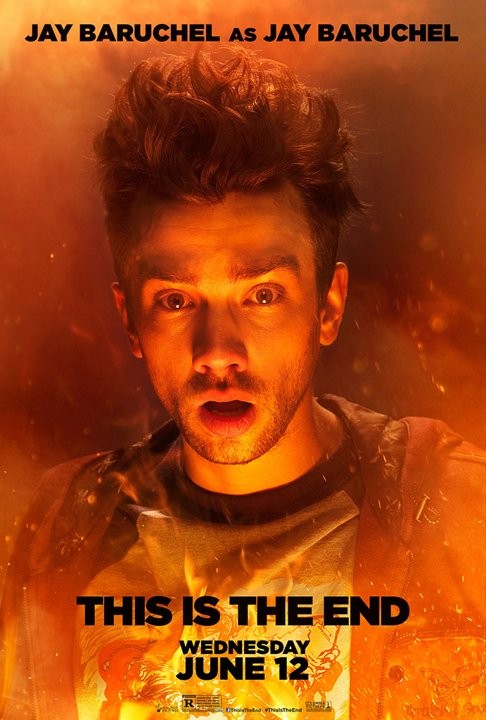The movie poster features an intense and dramatic image centered around actor J. Baruchel. At the top of the poster, in bold black lettering, it reads "J. Baruchel as J. Baruchel." Dominating the center is an image of J. Baruchel, a young Caucasian man with piercing eyes and dark hair styled straight up, showing a shocked expression on his face. His wide-open mouth highlights the intensity of the moment. He is dressed in a graphic t-shirt and a collared shirt, with a hoodie layered on top. Baruchel stands against a fiery backdrop, with embers and subtle flames rising up around him, casting an orange-red hue over his skin. The inferno behind and around him enhances the feeling of chaos and heat, as if he is engulfed in a hellish scene. Below the actor, towards the bottom of the poster, additional black text announces the movie title, "This Is The End," along with the release date, "Wednesday, June 12th." The poster also indicates that the film is rated R and is produced by Columbia Pictures.